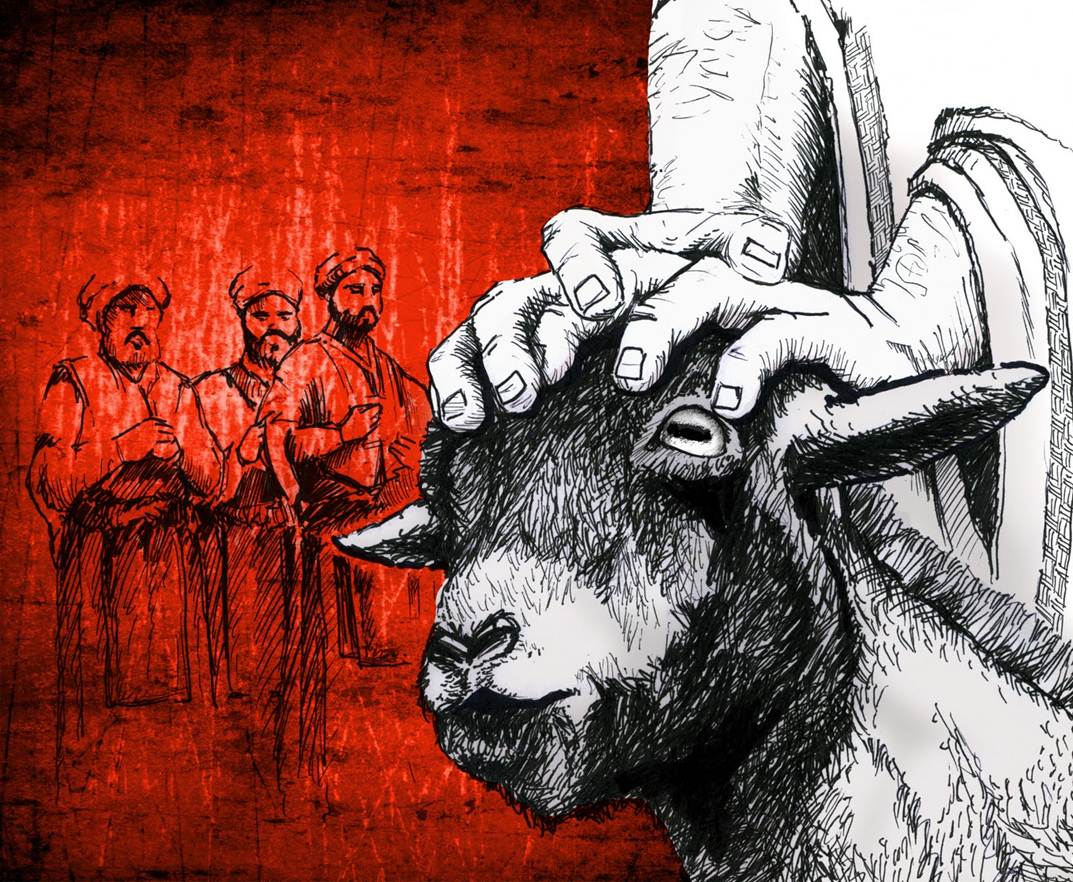This detailed illustration features a compelling juxtaposition of color and monochrome elements. The left side of the image is dominated by a deep red background with a grungy, streaky texture. Within this crimson expanse, three men, possibly the three wise men or figures involved in a religious ceremony, are depicted in black silhouettes. They are adorned with turbans and robes, each sporting mustaches and beards, and their hands are clasped or held in front of them, suggesting a formal or contemplative posture.

In stark contrast, the right half of the illustration transitions to a black and white scheme. Here, the central focus is the face of a lamb, oriented toward the left side of the frame. Two hands, appearing to be robed up to the wrists, press down gently on the lamb's head. These hands, positioned from the upper right to the center of the image, are prominent and add a solemn dynamic to the scene. The intricate detailing and thoughtful composition evoke a sense of ritualistic or shepherd-like care, bridging the colored and monochromatic halves into a singular, evocative narrative.